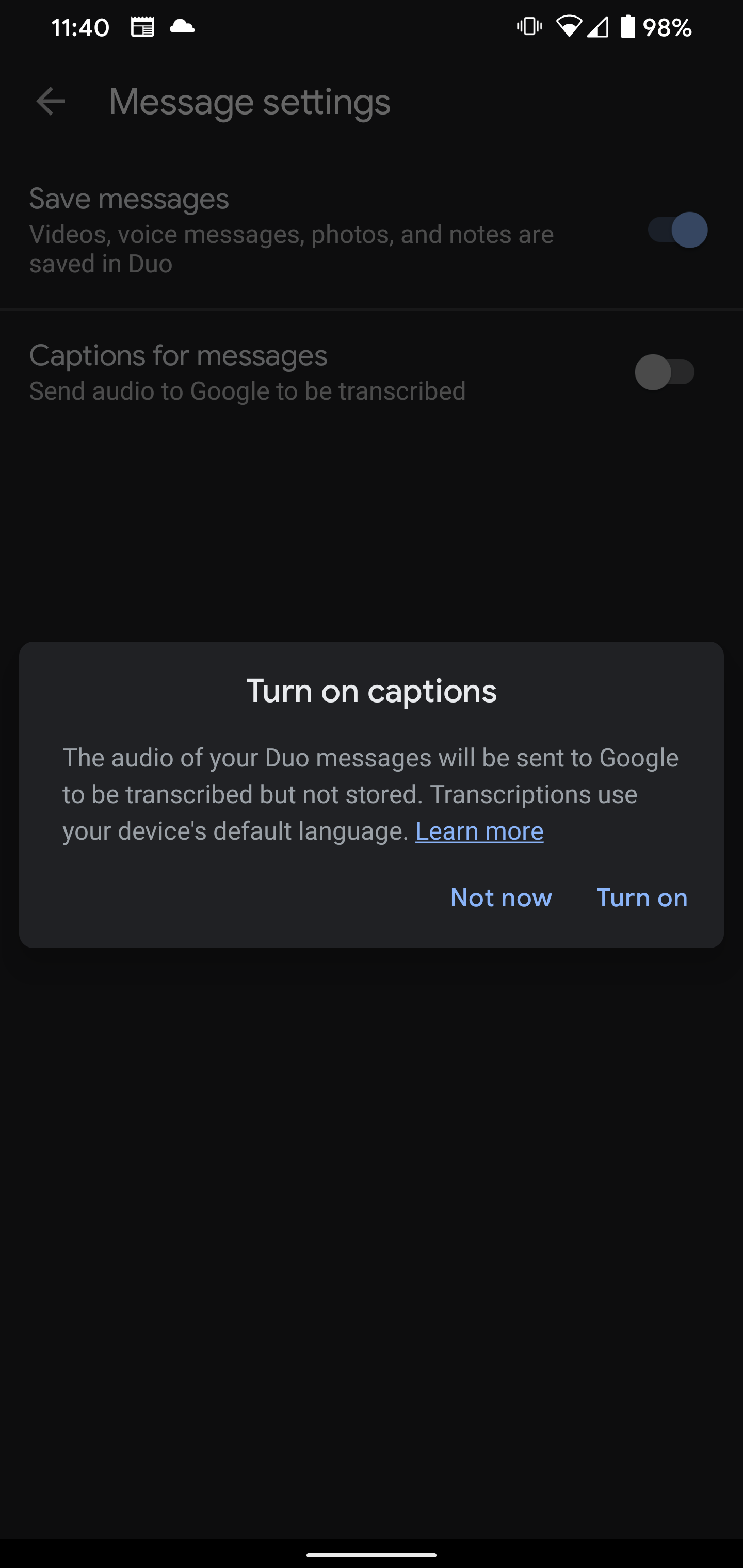The image showcases a smartphone screen displaying a mix of text and icons. At the top of the screen, the time is indicated as 11:40, along with various status icons including the Wi-Fi symbol and the battery percentage.

Lower on the screen, a pop-up notification prompts the user to "Turn on captions." The pop-up informs the user that audio from their Duo messages will be sent to Google for transcription, clarifying that the audio will not be stored. It also mentions that transcriptions will utilize the device's default language. The pop-up features three actionable buttons: "Learn more" in blue, "Not now," and "Turn on."

Higher up, the screen displays a back arrow and the heading "Message settings." Below this heading are various options, one of which is "Save messages." This option explains that videos, voice messages, photos, and notes will be saved in Duo. A blue indicator next to this setting suggests it is currently turned on. Another option titled "Captions for messages," which is explicitly noted as sending audio to Google for transcription, is shown as turned off.

The majority of the screen sports a black background with white text, accented by occasional blue text and buttons. The design includes a variety of icons typical of a smartphone interface, enhancing the overall detailed view of the screen's content.